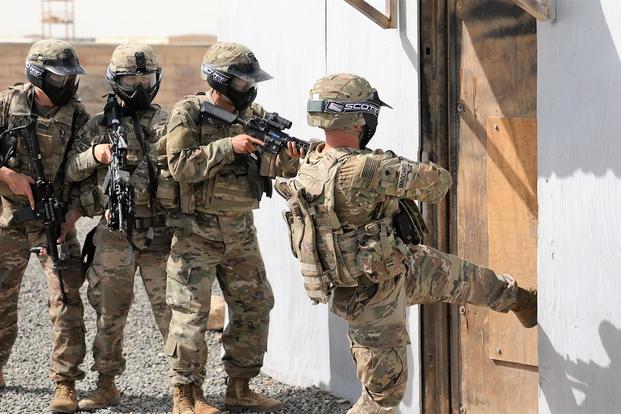The color photograph depicts four soldiers, likely Marines, in full camouflage gear, standing in front of a white plastered building with a dark brown wooden door. The ground is covered with gravel, and other cityscape elements are faintly visible in the background. All soldiers are equipped with helmets, face masks, camouflage jackets and pants, bulletproof vests, and tan work boots. They each carry automatic weapons.

The soldier at the forefront is actively kicking the door with his left leg. He has a name tag on his arm that appears to read "MACCARO." The second soldier is closely behind him, aiming his rifle directly at the door. The third soldier holds his weapon at a slight angle, while the fourth, who is partially turned towards the camera, keeps his rifle pointed towards the ground. This positioning and one soldier's acknowledgment of the camera suggest that the scene may be staged.

The arrangement of the soldiers and their focused readiness give the impression of a door-breaching mission, reminiscent of urban combat scenarios seen in conflicts such as those in Iraq.